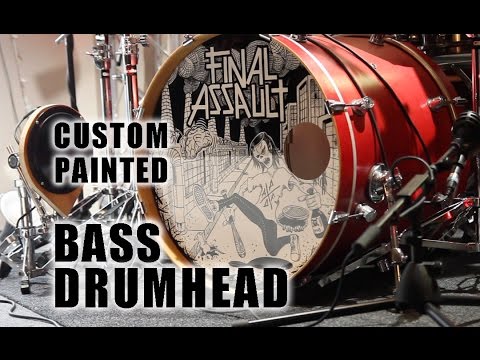This image features a red drum set with a custom-painted bass drum head prominently displayed, suggesting it's an advertisement for a drum customization service. The focal point is a large bass drum bearing the name "Final Assault" and a striking black-and-white illustration of a character with black hair and black pants, wearing a white shirt, and holding a bat and a drink, possibly in a city setting. Above this unique artwork, bold black text with a white glow reads "CUSTOM PAINTED BASS DRUMHEAD." Surrounding the central drum are other pieces of the drum set and some undetermined equipment, enhancing the overall impression that this service is tailored for bands or individuals seeking personalized drum designs.